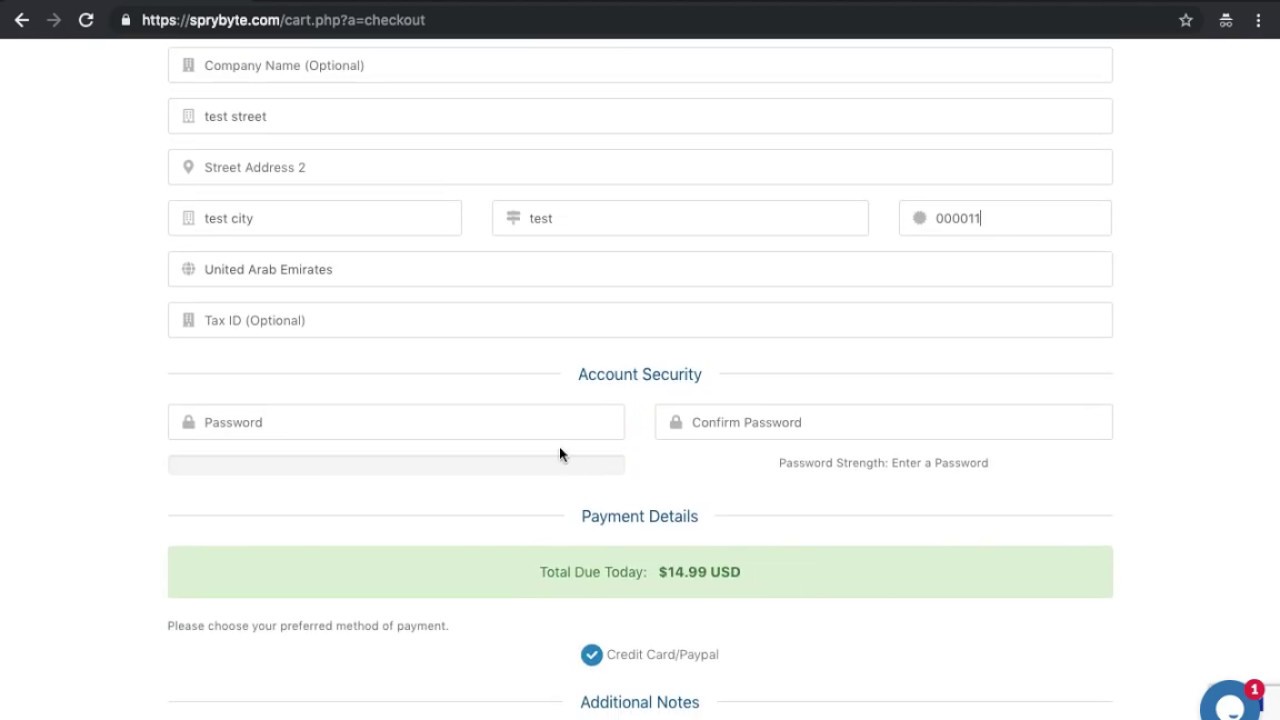The image depicts a black compound background featuring various white and gray elements. On the left-hand side, there is a prominent white arrow pointing to the left, accompanied by a gray arrow pointing to the right. A central oval shape, bordered in gray, contains multiple sections.

At the top left portion within the oval, a white line is present. Nearby are three small white circles arranged in a reflective manner. Within the oval, a pattern of rectangles extends from the left to the right. Adjacent to the gray border of the oval, a series of text fields are visible, each accompanied by descriptive labels.

The first label, displayed in gray, reads "Company Name" with a note indicating it is optional. Sequentially, the fields are labeled "Test Street," "Street Address 2," "Test City," and simply "Test." Another gray circle is marked with "000011," followed by "United Arab Emirates," and "Tax ID" (also noted as optional).

Further down, two fields denote the entry of passwords. Each field includes a gray lock icon for "Password" and "Confirm Password," along with a note on password strength. Labels towards the bottom read "Account Security" and "Payment Details." Just below, a green-highlighted text states "Total Due Today: $14.99 USD."